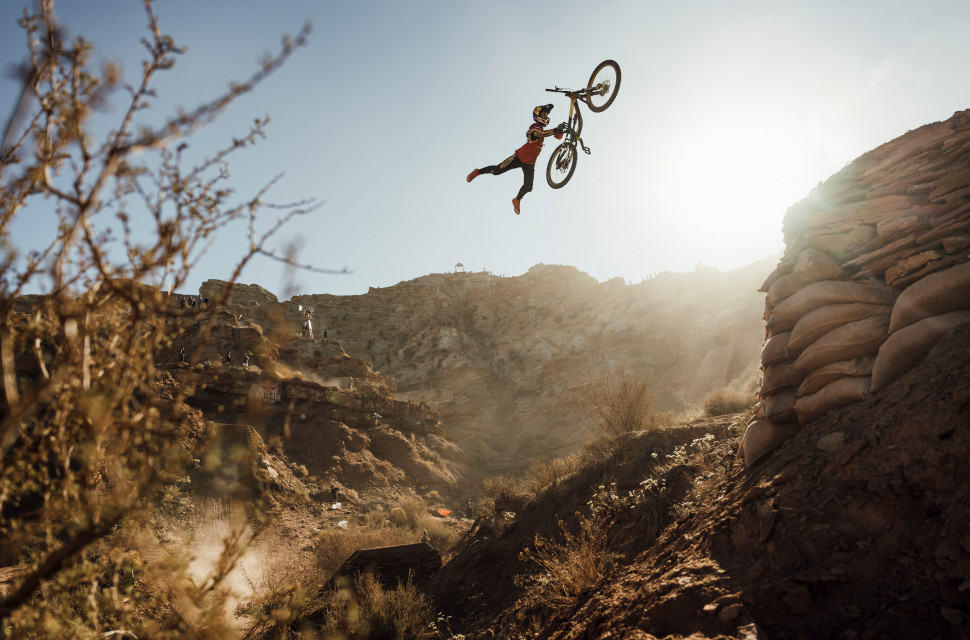A cyclist mid-air performs a daring bike split against a vivid blue sky backdrop. The scene unfolds in a rugged area featuring a small hill adorned with brown plants in the left foreground. The rider, clad in a red shirt and protective helmet, is captured gripping the seat of a predominantly black bike with striking yellow accents. To the right, an array of flat, stacked rocks, held in place by sandbags, forms a makeshift barrier reminiscent of a small canyon. The image encapsulates a thrilling moment of airborne action set amidst a diverse and textured landscape.